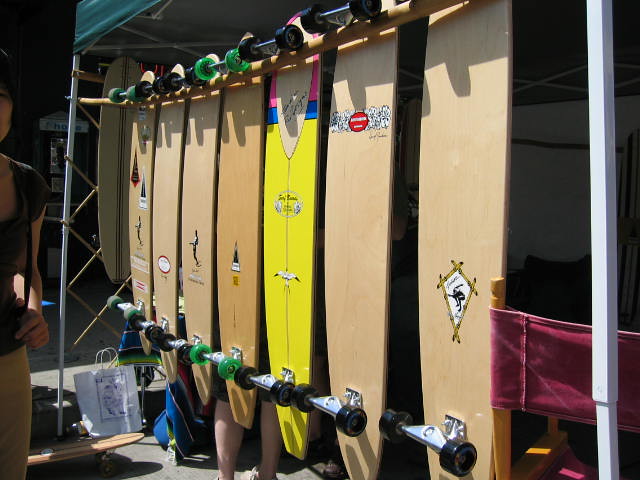The photograph captures a vibrant street fair scene, showcasing seven surf skateboards hanging on display under a green-topped pop-up tent. The skateboards are suspended from a horizontally fastened wooden pole, which is supported by silver metal posts on each side of the tent. Most of the skateboards feature a natural wood color with various stickers and logos on their undersides, making them unique. Among them, one skateboard stands out with its bright yellow base accented with pink and blue stripes, adding a splash of color to the display. The wheels of the skateboards are either black or green, with only one having green wheels. To the right, a maroon folding director's chair is visible, adding a casual element to the scene. On the left-hand side, part of a woman wearing a black t-shirt and short shorts is seen, her face partially visible along with her backpack straps. Additionally, behind the row of skateboards, a pair of legs and shoes peek out, suggesting another person in the background. The overall setup implies a street vendor selling these skateboards in an open, lively atmosphere.